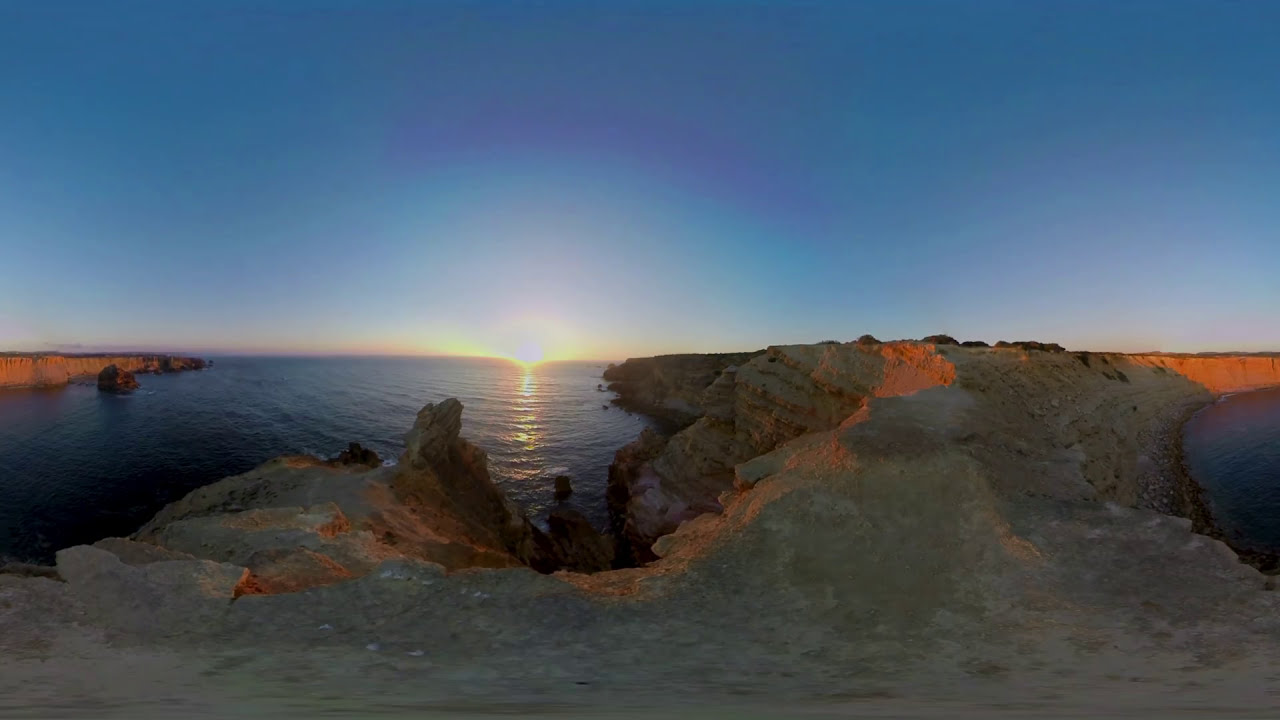The image captures a rugged coastal cliff during what appears to be a sunrise or sunset, given the presence of a yellow-orange light from the sun. The scene is devoid of people, emphasizing its untouched, natural state. The cliff is characterized by sheer drops and craggy, rocky surfaces, enhancing the remote and wild atmosphere. On both sides, the cliff extends into the water, creating a dramatic juxtaposition between the land and the open ocean. In the foreground, waves crash against large rocks and boulders in the water, adding movement and texture to the scene. The sky above is clear, transitioning from a purplish haze near the horizon where the sun sits, to a deeper blue higher up. The reflection of the sun on the water and the cliff adds a warm, orange-ish glow to the otherwise gray and brown rocky landscape. The area looks inhospitable with its steep drops and dry sand, not suited for leisurely activities like sunbathing.